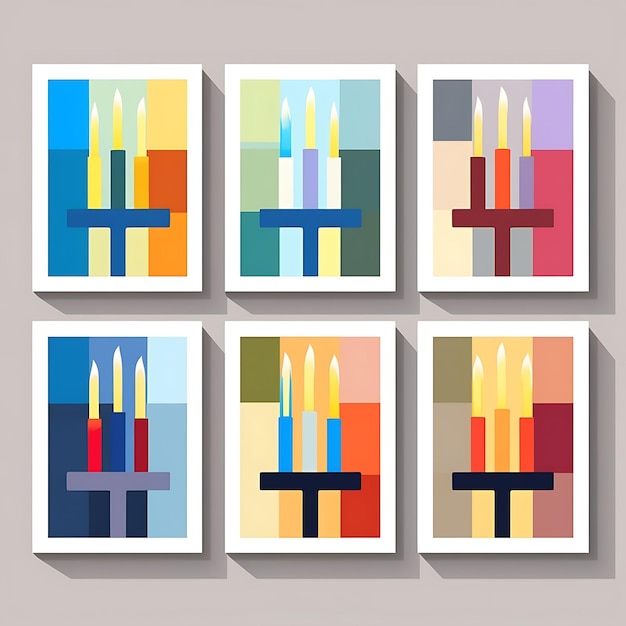The image showcases an abstract artwork mounted against a light gray wall, featuring six rectangular pieces arranged in two rows and three columns. Each piece of artwork is identical in composition but varies in color schemes, framed by white borders. The artwork depicts three vertical, candle-like figures situated on a pedestal in the shape of a 'T,' with each middle "candle" appearing taller than the ones on either side. Various shades of blue, along with combinations of green, orange, red, pink, and yellow, dominate the color palettes of these geometric blocks. Shadows cast on the wall suggest that the lighting is coming from the upper left-hand side. The designs are composed of sharp lines and solid geometric shapes, with detailed color blocks that include shades of beige, deep orange, maroon, and teal. The overall simplicity and precision in the shapes lend a cohesive yet vibrant visual effect to the artwork.